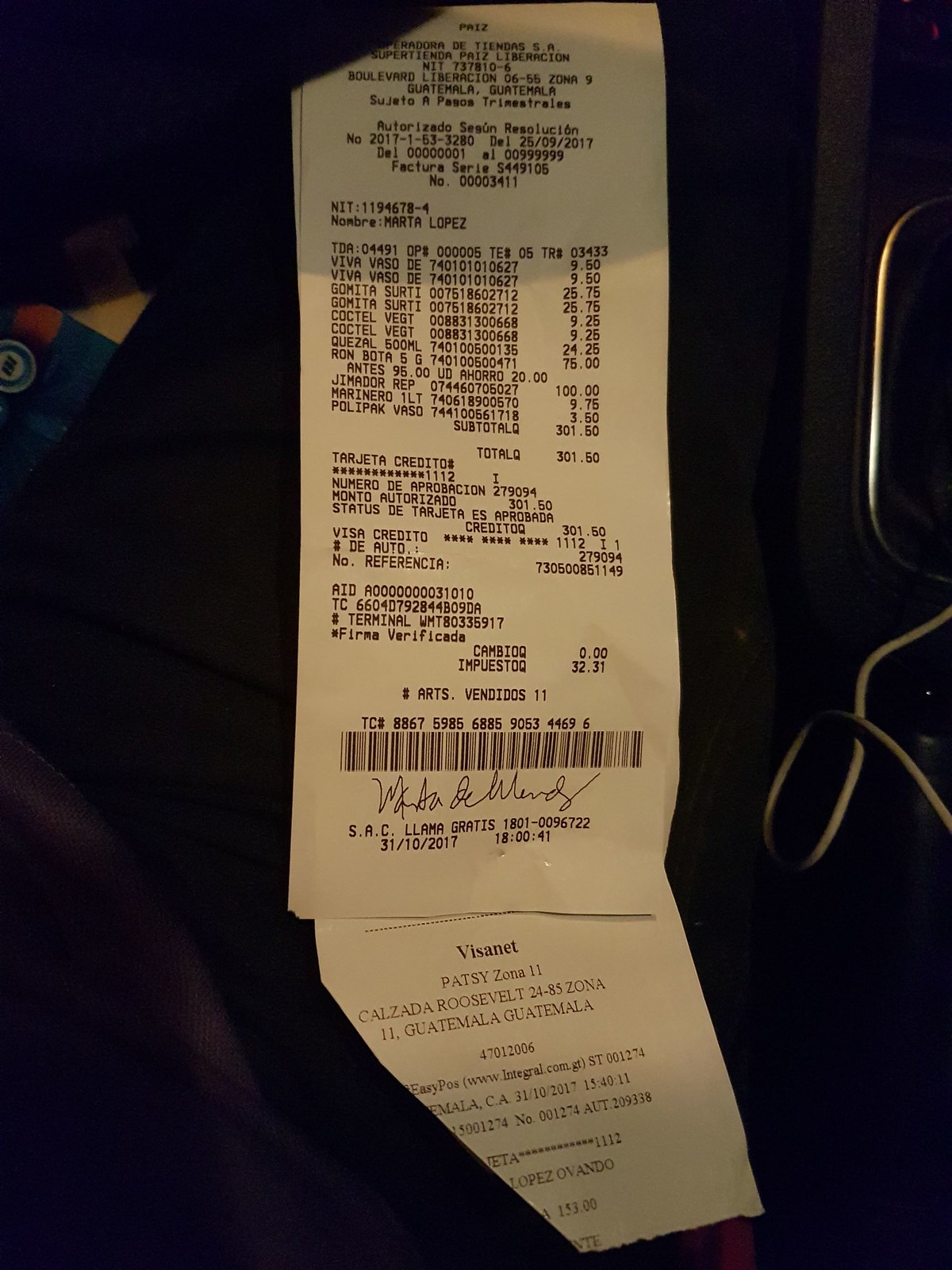A detailed photograph captures a long receipt printed on white paper with black ink, originating from an establishment in Guatemala. The receipt, totaling $301.80, features a signature at the bottom and is placed against a royal blue fabric backdrop. Sunlight illuminates the lower portion of the receipt, casting shadows over the upper part. To the right of the receipt, a small metal object is visible, adding an intriguing element to the composition.